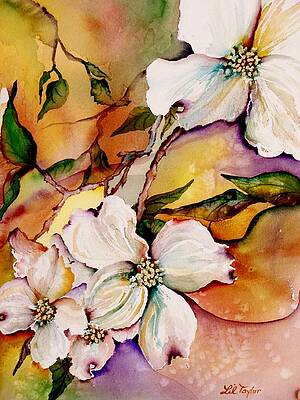The image is a painting of white flowers, prominently featuring artist Lil Taylor's signature in brown cursive in the lower right corner. This vertically aligned, smaller-sized, rectangular artwork has no visible border and gives the impression of being either a watercolor or acrylic on canvas, though it might also be a print. The composition is well-lit, showcasing an array of colors in the background such as greens, browns, pinks, purples, peach-orange, and the occasional swirl of light brown through the flowers. 

The flowers, mostly concentrated towards the upper right corner and center, are characterized by their four to five white petals adorned with subtle light brown streaks and purple spots on the tips, encapsulating visible little seeds in the middle. The background, particularly in the upper left and lower right, blends a mixture of brown, green, and peachy hues that could represent leaves, dirt, or simply an abstract color palette. The depiction of leaves appears more concentrated around the middle, with hues ranging from green to orange, often featuring pointed tips.